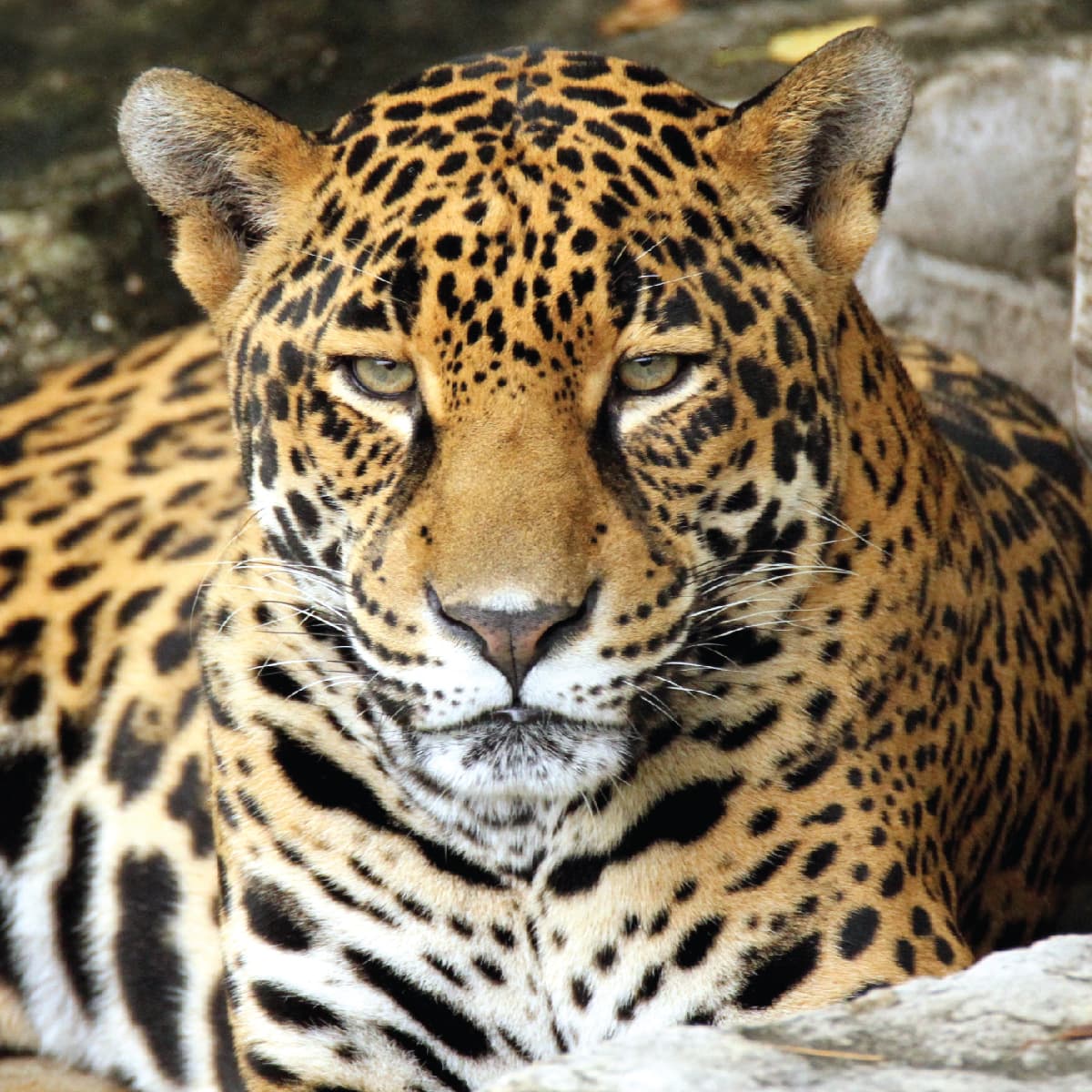The image captures a leopard in a perfectly square frame, lying down amidst a backdrop of rocks, possibly within a cave or shaded area. The leopard is staring directly into the camera with a menacing, half-closed gaze, giving it an intense and focused look. Its golden fur is adorned with numerous black spots, particularly visible on its head. The leopard sports green eyes highlighted with white under-eye markings that resemble eye shadow. Its nose and chin feature white patches, complementing the white regions on its belly. The ears are outlined in black, with a touch of white hair inside, and its white whiskers are interspersed with a few black ones. The animal's head is held up alertly, adding to its vigilant demeanor.